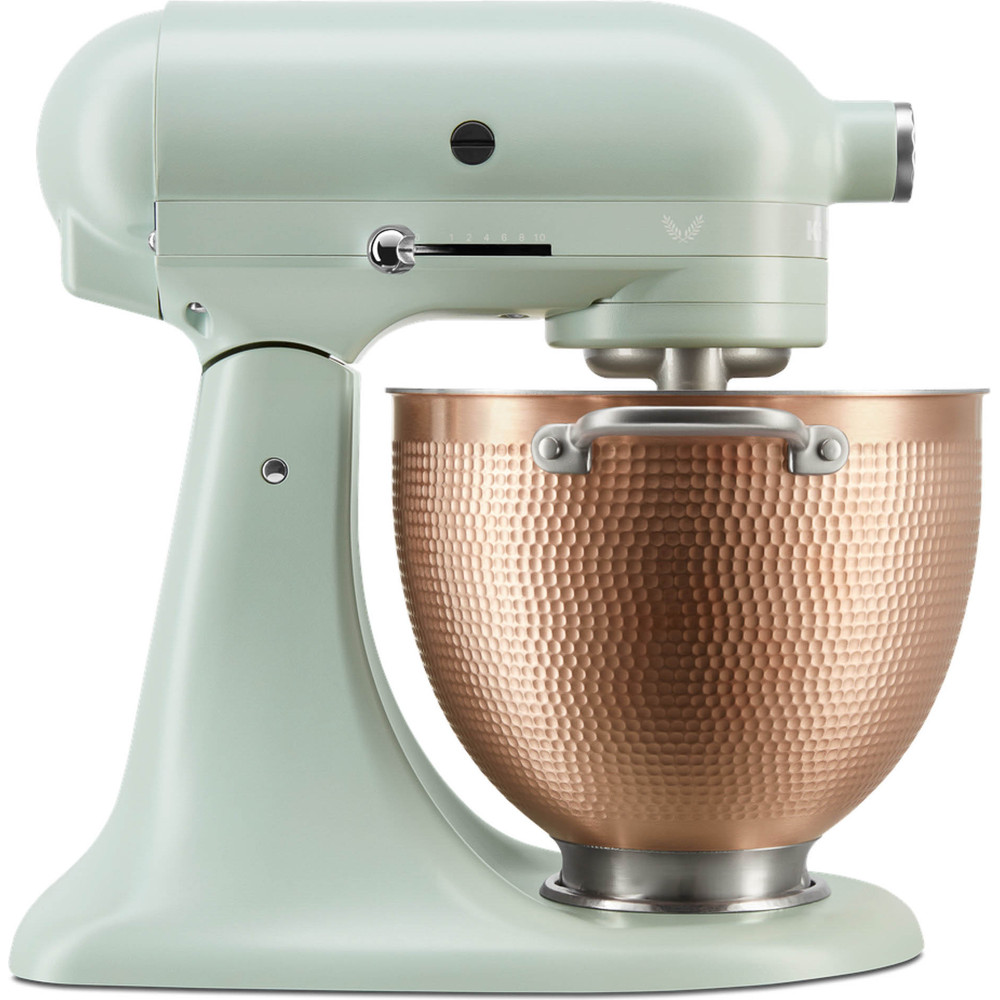This photorealistic image captures a stand mixer set against a blank white background. The body of the mixer features a pale green-gray color, resembling a light sage or faded mint green, and is shown in a side profile facing to the right. Prominent in the image is its hammered copper mixing bowl, adorned with a distinctive textured pattern of tiny dots and circles. The copper bowl is equipped with a silver handle near the top and a silver base that fits into the mixer's broad, sleek steel base. The mixer's structure elegantly narrows upward before expanding again into its standard cylindrical form. Silver accents—including a stainless steel dial on the front, silver bolts around the mixer, and a stainless steel knob linked to a black slider marked with the numbers 1, 2, 4, 6, 8, and 10 in white text—add to its visual appeal. Additionally, the top of the mixer arm displays a cut black bolt and what seems to be a tiny white butterfly stamp. Concluding the mixer’s right-hand view, a silver metal mixer attachment connects seamlessly into the bowl.